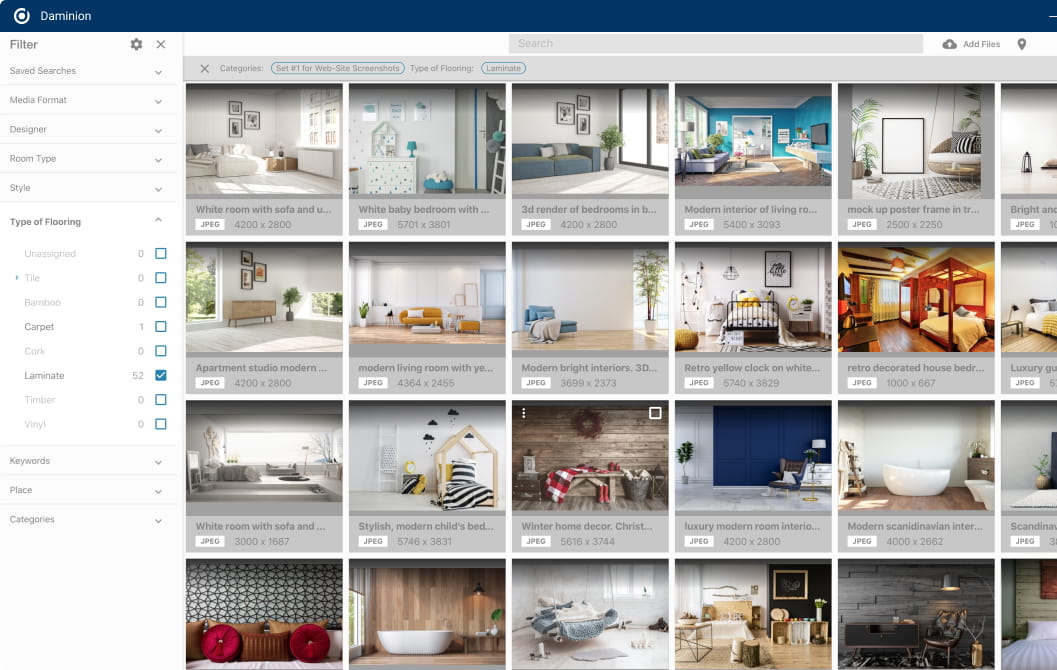The image showcases a digital interface for a website named Damminion, focused on sourcing various interior room photographs. Prominently on the right side of the screen, there are multiple filter options and tabs available for refining searches—these include saved searches, media format, designer, room types, style, and types of flooring. The "types of flooring" filter is currently expanded, revealing additional object options. The selected flooring type is laminate, out of a total of 52 available types. Under the flooring filter, there are several categories: unassigned, tile, bamboo, carpet, cork, laminate, timber, and vinyl. Further down, there are tabs for additional filters such as keywords, places, and categories. The central area of the screen displays a grid of images arranged in a 5x4 format, showing interior room samples. It appears that a sixth image on the right edge has been partially cut off. All displayed images are in JPEG format.